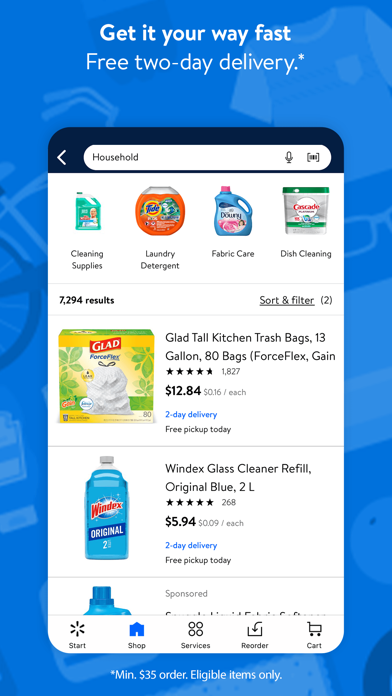This is an image of an advertisement for a household product application, featuring a visually appealing blue background in various shades. At the top of the image, a bold white headline reads, "Get it your way — fast, free two-day delivery." An asterisk at the bottom of the image corresponds to a footnote stating, "Minimum $35 order, eligible items only."

The central portion of the image showcases a virtual search interface labeled "Household," including icons for voice search and barcode scanning. Below the search bar, categories like "Cleaning Supplies," "Laundry Detergent," "Fabric Care," and "Dish Cleaning" are listed, indicating the breadth of available products. The search results indicate a substantial inventory, with "7,294 results" displayed prominently.

The interface offers sorting and filtering options, enhancing the user experience. Three product descriptions are visible, emphasizing the range and pricing of the items. 

The first product is "Glad Tall Kitchen Trash Bags, 13 Gallon, 80 Bags, ForceFlex, Gain," priced at $12.84, which breaks down to approximately $0.16 per bag. This product boasts tags indicating "Two-Day Delivery" and "Free Pickup Today."

The second product is "Windex Glass Cleaner Refill, Original Blue, 2 Liters," priced at $5.94, also featuring "Two-Day Delivery" and "Free Pickup Today" options. 

These detailed descriptions highlight the convenience and affordability of the products, reinforcing the ad's promise of fast and free delivery for essential household items.